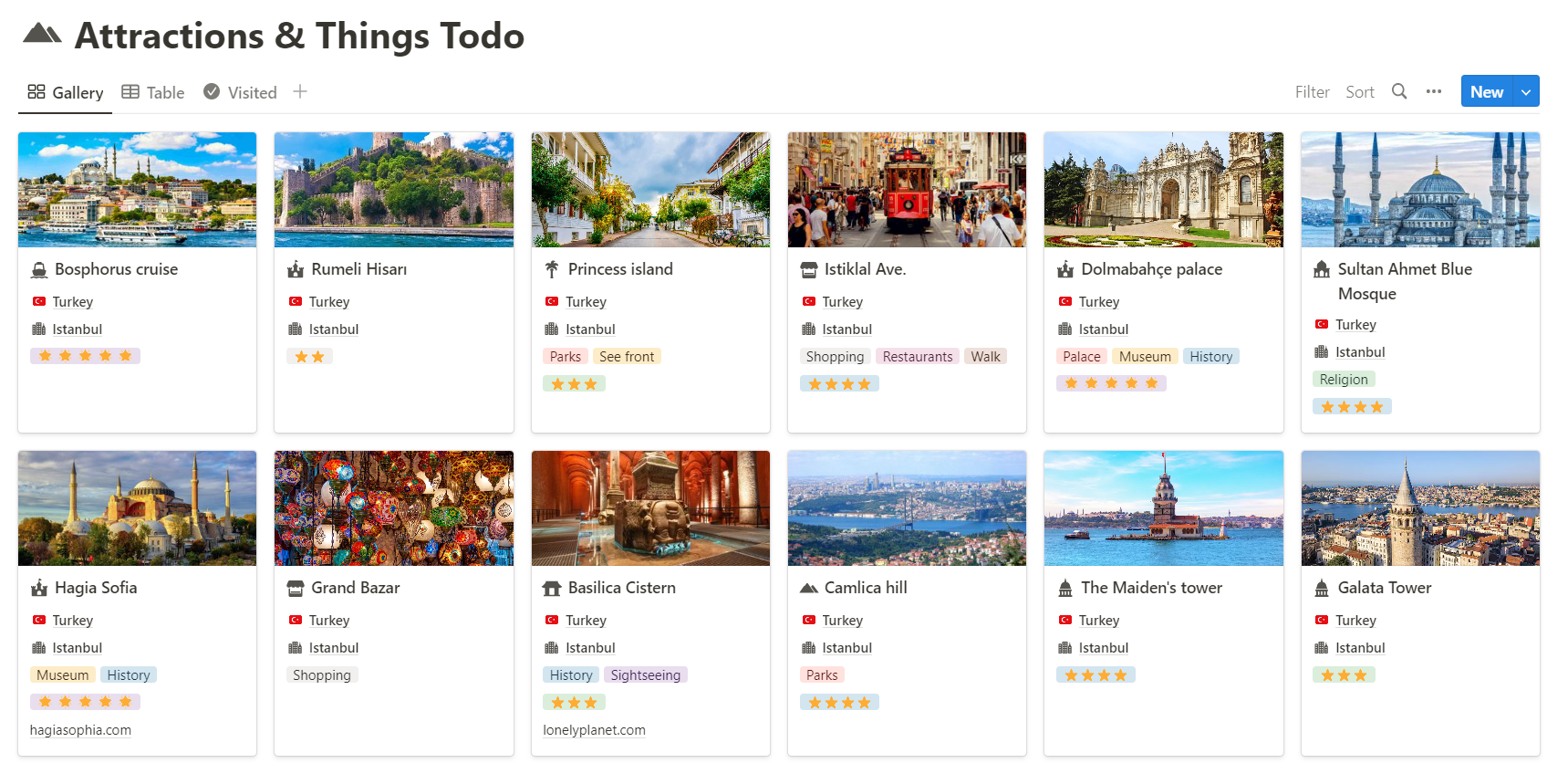The image showcases the top attractions and things to do, all consolidated into a single-word category titled "to do." Beneath this category, there are three tabs: "gallery," "table," and "visited," with the "gallery" tab currently open. The attractions listed include:

1. **Bosphorus Cruise, Istanbul, Turkey**: Rated five stars.
2. **Rumeli Hisari, Istanbul, Turkey**: Rated two stars.
3. **Princess Island, Istanbul, Turkey**: Parks and seafront area, rated three stars.
4. **Istiklal Ev, Istanbul, Turkey**: Shopping and restaurants area, rated five stars.
5. **Hagia Sophia, Istanbul, Turkey**: A historical museum associated with the website hagiasophia.com, rated five stars.
6. **Grand Bazaar, Istanbul, Turkey**: Shopping area, not rated.
7. **Basilica Cistern, Istanbul, Turkey**: Historical sightseeing spot, rated three stars, associated with lonelyplanet.com.
8. **Kamalaka Hall, Turkey**: Mentioned under parks.
9. **Maiden's Tower, Turkey**: Rated four stars.
10. **Galata Tower, Istanbul, Turkey**: Rated three stars.
11. **Sultanahmet Blue Mosque, Istanbul, Turkey**: Noted for its religious significance.

The attractions span a variety of interests including cruises, historical sites, shopping districts, parks, seafronts, and religious edifices, offering a comprehensive guide to Istanbul's must-see destinations.